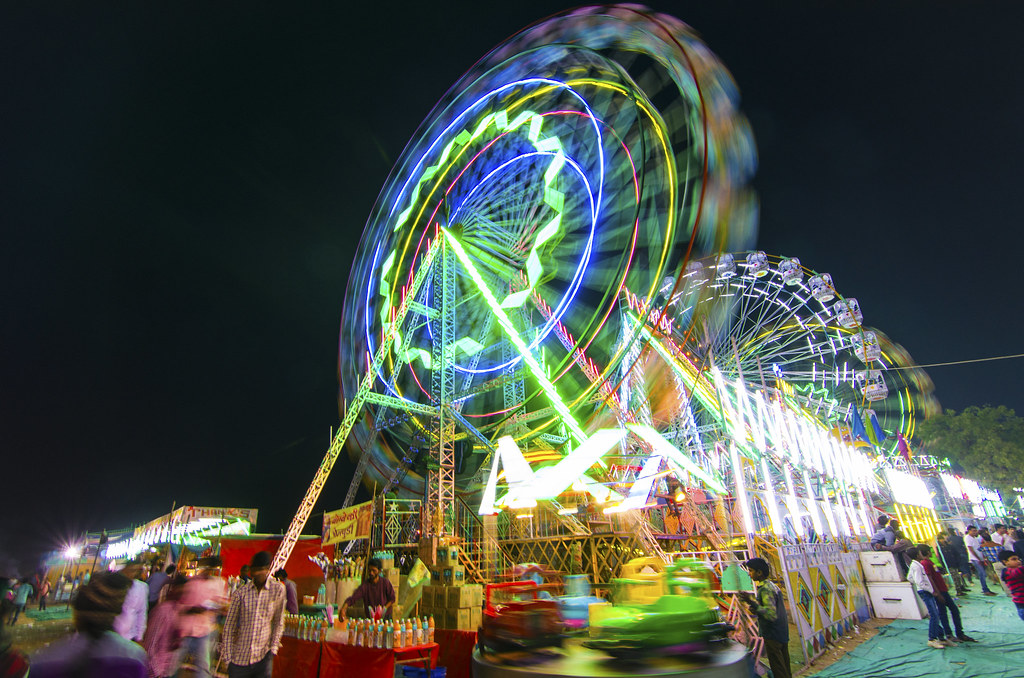This photograph captures a vibrant nighttime carnival scene with a dynamic array of attractions and a bustling crowd. Centered prominently is a large green Ferris wheel, adorned with colorful neon lights in hues of green, yellow, and blue. The Ferris wheel is captured in motion, creating a blurred effect that conveys its swift rotation. Surrounding this main Ferris wheel are two additional, smaller Ferris wheels, also illuminated with vibrant neon lights in shades of purple, yellow, and green, adding to the festive atmosphere. The entire scene is bathed in the deep blue of the night sky, enhancing the vividness of the neon lights. In the foreground, various booths and rides, including a spinning ride with rotating cars, contribute to the lively ambiance. The photo depicts numerous people scattered around the fairgrounds, walking and enjoying the attractions, giving the image a dynamic and bustling feel.